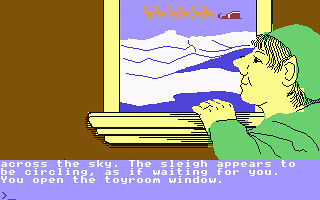This image appears to be a still from an older, pixel-art style video game, resembling a quaint scene from a children's book. It features a yellow-skinned elf-like creature with stringy black hair, pointed ears, a peculiar nose, dressed in green attire with a matching green hat. The elf stands to the right of the frame, gazing out of a pale yellow window set in a dark brown wall.

Beyond the window, the backdrop showcases snow-covered glaciers and patches of blue water, accompanied by Santa Claus's red sleigh pulled by six light tan reindeer. The sleigh is depicted mid-flight, circling in the sky as if waiting, with the text beneath the scene reading in white text against a purple background: "Across the sky, the sleigh appears to be circling as if waiting for you. You open the toy room window."

The entire scene, captured in a style reminiscent of artwork created in Microsoft Paint, evokes a charming, nostalgic feel, further emphasized by the pixelated zigzag patterns typical of early digital art.